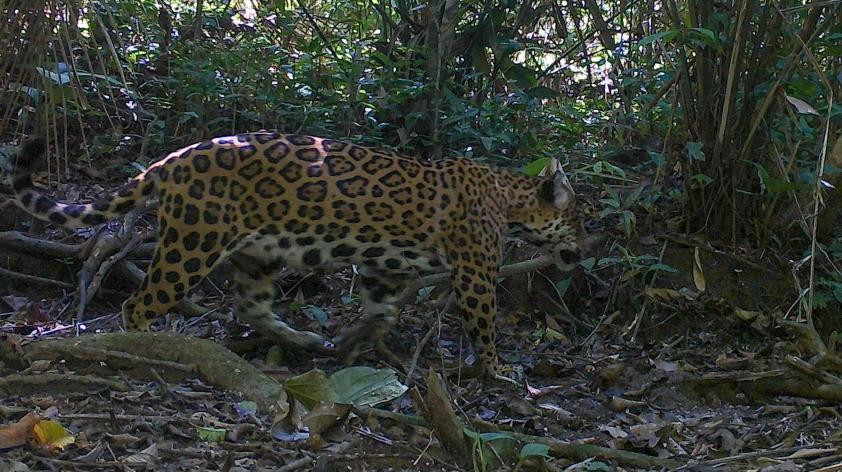In this image, we see a large wild cat, likely a cheetah or leopard, roaming through its natural habitat. The setting is a dense, lush forest area with a mix of green and brown leaves covering the ground along with various shrubs and twigs. The scene is dappled with glimpses of sky filtering through the thick canopy of trees. The wild cat, distinguished by its golden coat adorned with dark spots and markings, appears to be either on the prowl or in mid-stride, taking up a significant portion of the frame. The surroundings are a vibrant mix of natural foliage and mulching leaves, emphasizing the untamed beauty of this wilderness area.